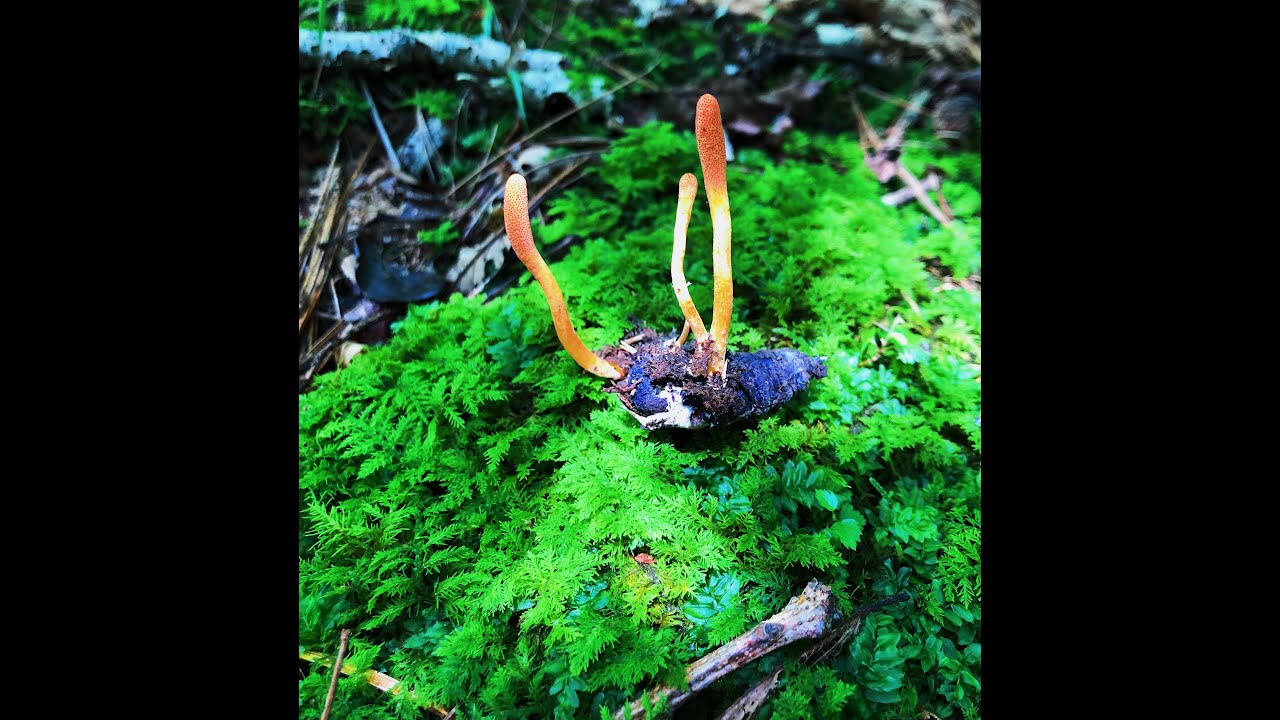In the center of this forest scene, amidst lush green ferns and leafy moss, stands a curious and visually striking organism. The background features blurred trees and branches, but the focus is drawn to a peculiar entity that appears both plant-like and otherworldly. Rising from a mottled blue and purplish base are three spindly, tentacle-like strands. These tendrils exhibit a gradient of colors, starting with a light yellow at the bottom and transitioning to a vibrant orange and red at the tops, reminiscent of a candy corn pattern. This enigmatic fungus or plant-like figure, with its distinctly vivid tendrils, creates a surprising contrast to its surrounding earthy foliage and commands the viewer's attention in this captivating nature photograph.